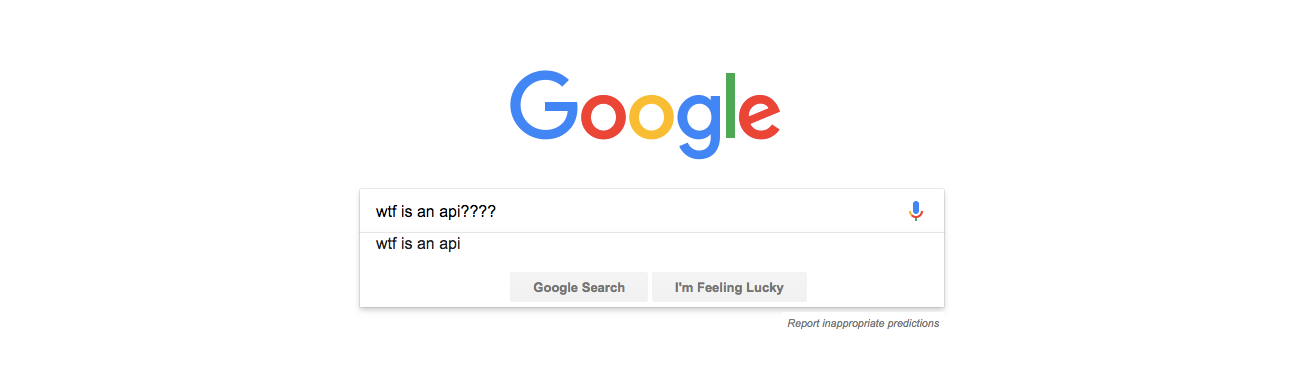The image depicts a minimalistic Google search bar interface, characterized by Google's distinctive, multicolored logo prominently displayed at the top. At the center of the search bar, a user-typed query reads, "WTF is an ABI????," punctuated with four question marks, reflecting a sense of urgency or confusion. Below the typed query, a suggested search appears, offering additional guidance or potential related queries for the user's consideration. To the right of the search bar, an icon of a microphone is visible, indicating the option for voice search, allowing users to speak their queries instead of typing. Positioned underneath the search bar are two standard Google search buttons: "Google Search" and "I'm Feeling Lucky," providing users with different navigation choices for initiating their search.